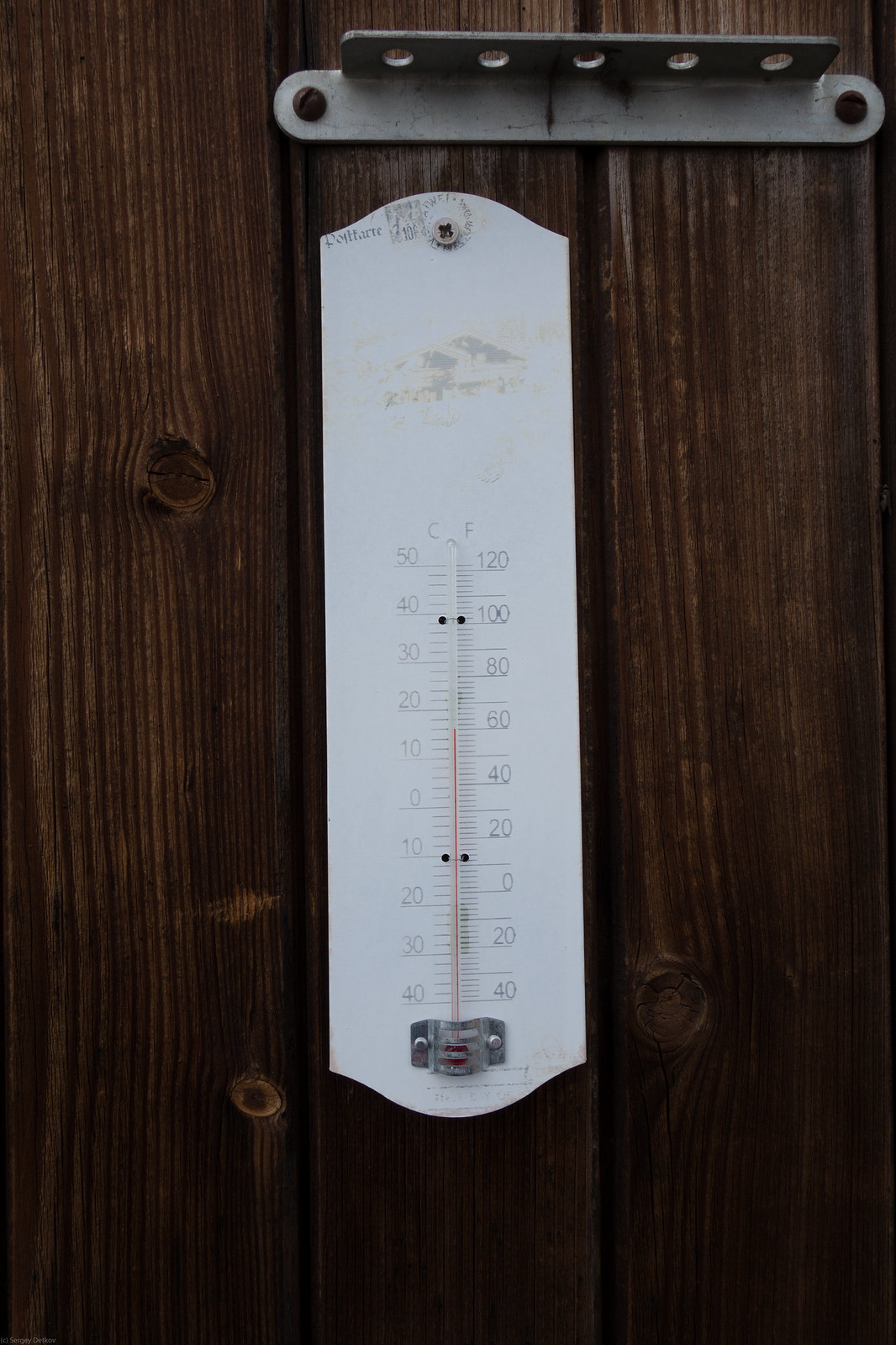A white thermometer is prominently mounted on a richly grained, dark wooden surface, with the vertical lines of the wood adding texture and depth to the scene. The thermometer is securely fastened at the top by a white screw, ensuring its stability. The device shows signs of wear, as indicated by its faded lettering. The left side of the thermometer is marked with the letter 'C' and has a scale ranging from -40 to 50 degrees Celsius, increasing from bottom to top. On the right side, it is labeled 'F' and displays temperatures from -40 to 120 degrees Fahrenheit in the same bottom-to-top progression. The red mercury line of the gauge, a crucial indicator of temperature, currently hovers just above the 10-degree mark on the Celsius scale and about 15 degrees on the Fahrenheit scale. The bottom of the thermometer is securely held in place by a silver clasp, which is fastened with screws on either side, ensuring the device is firmly attached to its base. Above the thermometer, a metallic bracket or piece is affixed to the wood, featuring dark screws on either side and an extension with five holes, adding an industrial element to the rustic wooden backdrop.